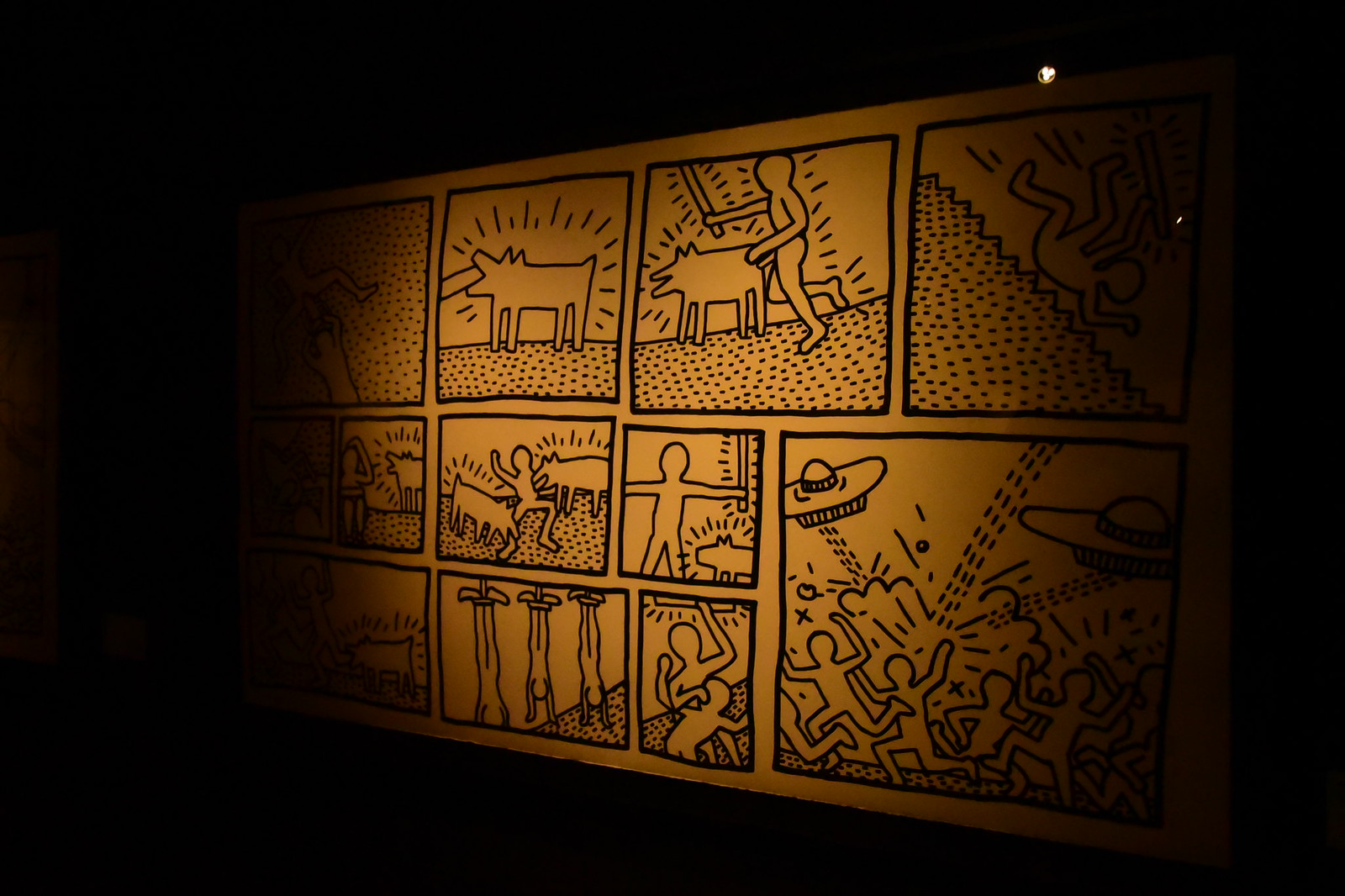The image features a comic book style drawing with a gold background and black illustrations, divided into several squares. Each panel depicts dramatic and chaotic scenes. In the top left, a dog is eating something, surrounded by motion lines. Next, a figure appears to be spanking or interacting aggressively with a dog, though the exact nature of the interaction is unclear. To the right, a man is depicted fighting off a pack of dogs or pigs. Another panel seems to be fading, showing people or animals tumbling down a hill. A prominent larger square at the bottom right displays people running around with a sombrero spinning in the air. An additional chaotic scene shows a spacecraft bouncing off the Earth, alarming nearby people, with another spaceship visible to the right. There are also cryptic symbols on the horizon, resembling an X, a Q, and an O. The overall composition has a dark undertone with intense, possibly violent interactions, all set against the same gold background with black shadow effects.